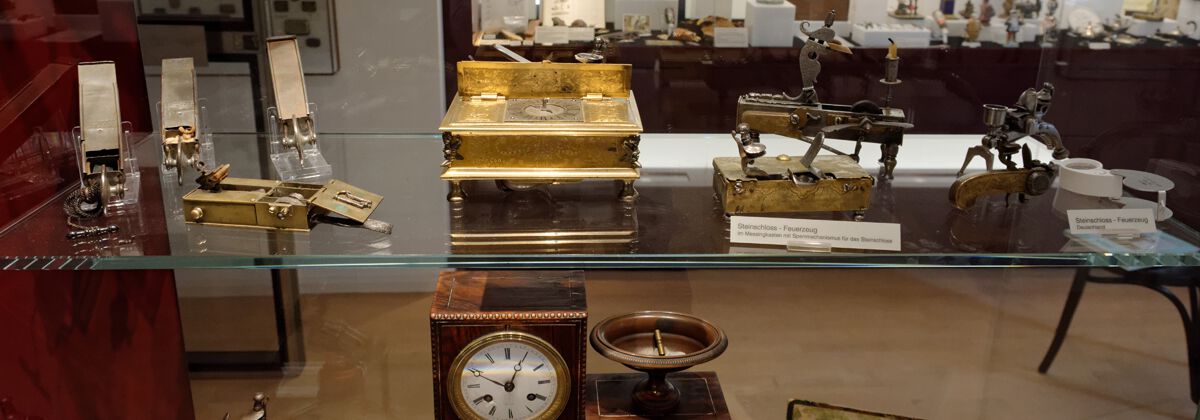This color photograph captures an intricately arranged museum showcase, highlighting a collection of historic artifacts. The display features a smooth tan floor and a background of wooden and glass cases filled with numerous items. Central to this image is a prominent glass shelf encased in glass on three sides and wood on the left, creating the illusion of a floating surface. 

Atop this glass table lies a curated selection of brass and wooden objects. Dominating the center is a small golden box with four legs and an opening mechanism, bearing what appears to be a clock face. Surrounding it are various mechanical devices, including three similar rectangular brass objects, possibly old cigar lighters with little wicks and strikers, and an item with visible gears on the right, which may be another clock or a different intricate mechanism.

Below this glass shelf, a wooden box houses a clock, easily visible through the glass. Beside it sits another item, perhaps a wooden or brass bowl on a stand, or a weighing machine. Accompanying these antiquities are white cards likely identifying each piece, though the text is illegible in the photograph. The sophisticated array of these metallic and wooden artifacts, possibly dating back to the 1800s, along with the intricate setup of the museum environment, conveys a sense of historical richness and meticulous preservation. The background also showcases another display across the hall, hinting at the expansive collection in the museum.